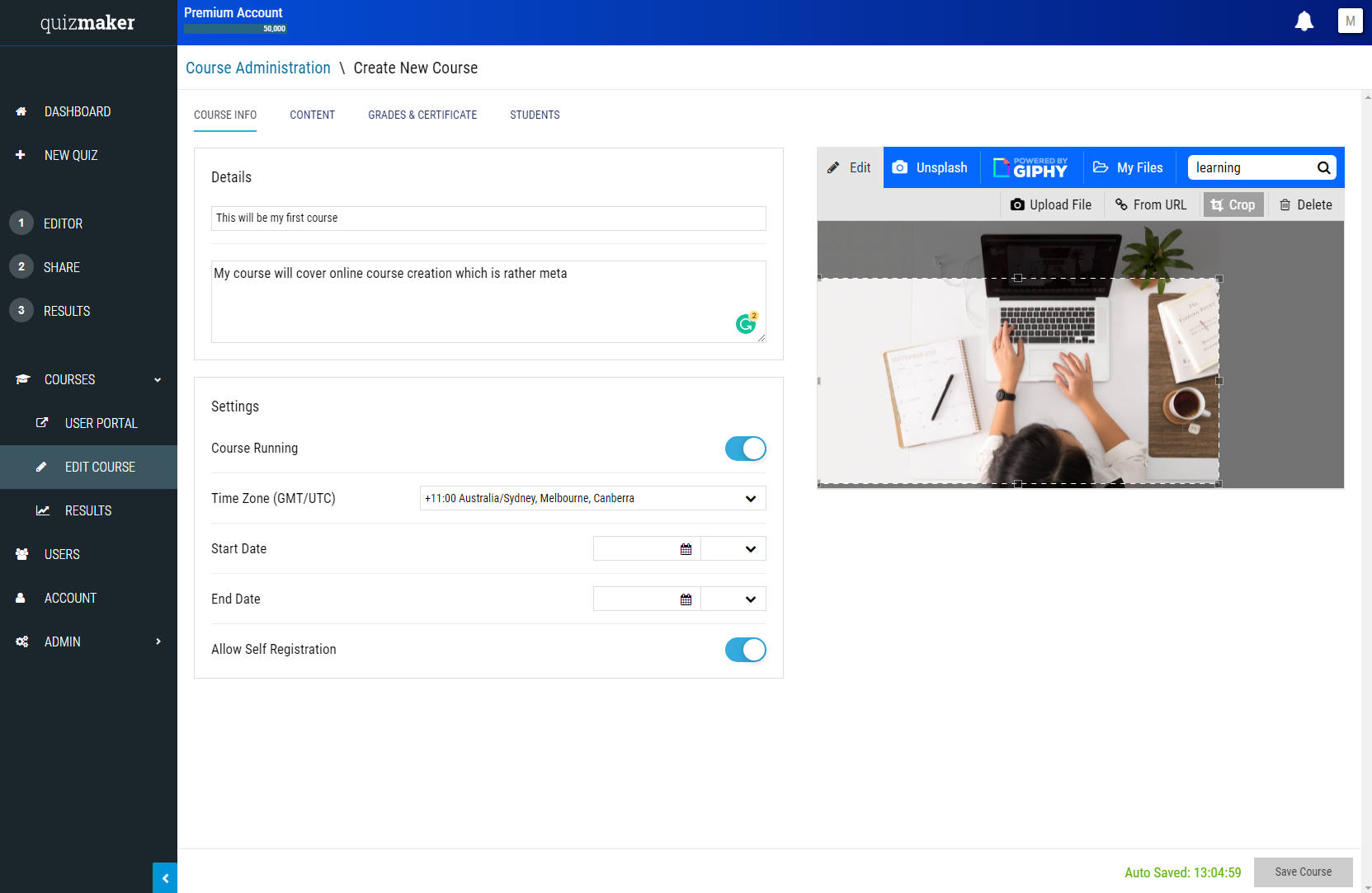The image showcases a digital interface for an online course creation platform called Quidmaker. At the top of the screen, there's a dark blue border featuring a "Premium Account" label and a notification bell on the right side. In the center of this border, there's a white square with the letter "M" inside it.

On the far left, there is a vertical menu that includes options such as "Course Administration," "Create New Course," "Course Info," "Content," "Grades and Certificates," and "Students." Below the menu, there is a section labeled "Details" alongside a text box containing the phrase "This would be my first course." Further down, another text box states, "My course will cover online course creation, which is rather meta." The word "meta" appears blurry and small.

Further down the interface, there is a "Settings" section detailing "Course Running Time Zone (GMT/UTC)." There are also input fields for "Start Date" and "End Date," each equipped with a calendar icon and a drop-down menu for selecting dates.